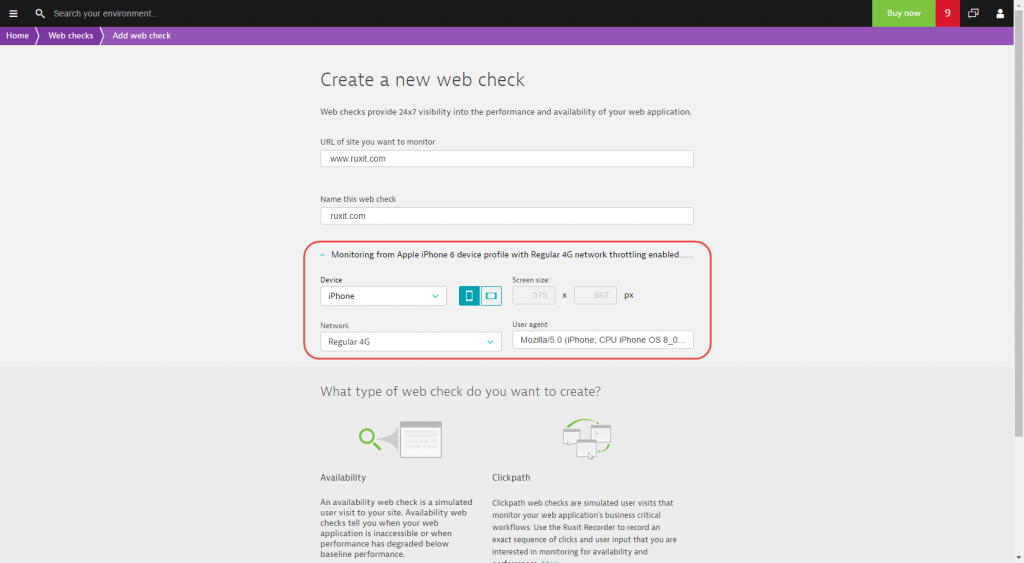Here's a detailed and cleaned-up descriptive caption for the image:

---

At the top of the screenshot, a small black banner is visible with three lines, representing a menu icon. On the left side, there is a search bar accompanied by a search icon, along with the text, "Search your environment." Below this, a purple banner is displayed with three tabs labeled: "Home," "Web Checks," and "Add Web Check."

The remaining area of the page has a white background. The first prominent line reads, "Create a new web check," in large gray letters. Following a space, there is a smaller line of text that states, "Web checks provide 24-7 visibility into the performance and availability of your web application."

Next, there is a prompt, "URL of site you want to monitor," followed by a rectangular input box containing the entry "www.rexit.com," indicating the user intends to monitor this site. Below this is another prompt, "Name this web check," with the name "rexit.com" entered in the adjacent box.

A distinct rectangular box with a red outline and gray interior contains small gray text at the top, which reads, "Monitoring from Apple iPhone and device profile with regular 4G network throttling enabled." A subsequent input box labeled "Device" has the entry "iPhone."

Two icons representing orientation choices—portrait and horizontal—are displayed, with the portrait option selected. The screen size section includes two input boxes for specifying dimensions. There is a dropdown box for selecting the network type.

Further down, there is a rectangular box labeled "User Agent," where the entry "Mozilla 5.0 (iPhone; CPU iPhone OS 8_0 like Mac OS X)" is typed in. The remaining portions of the screen contain additional information related to availability and click path settings.